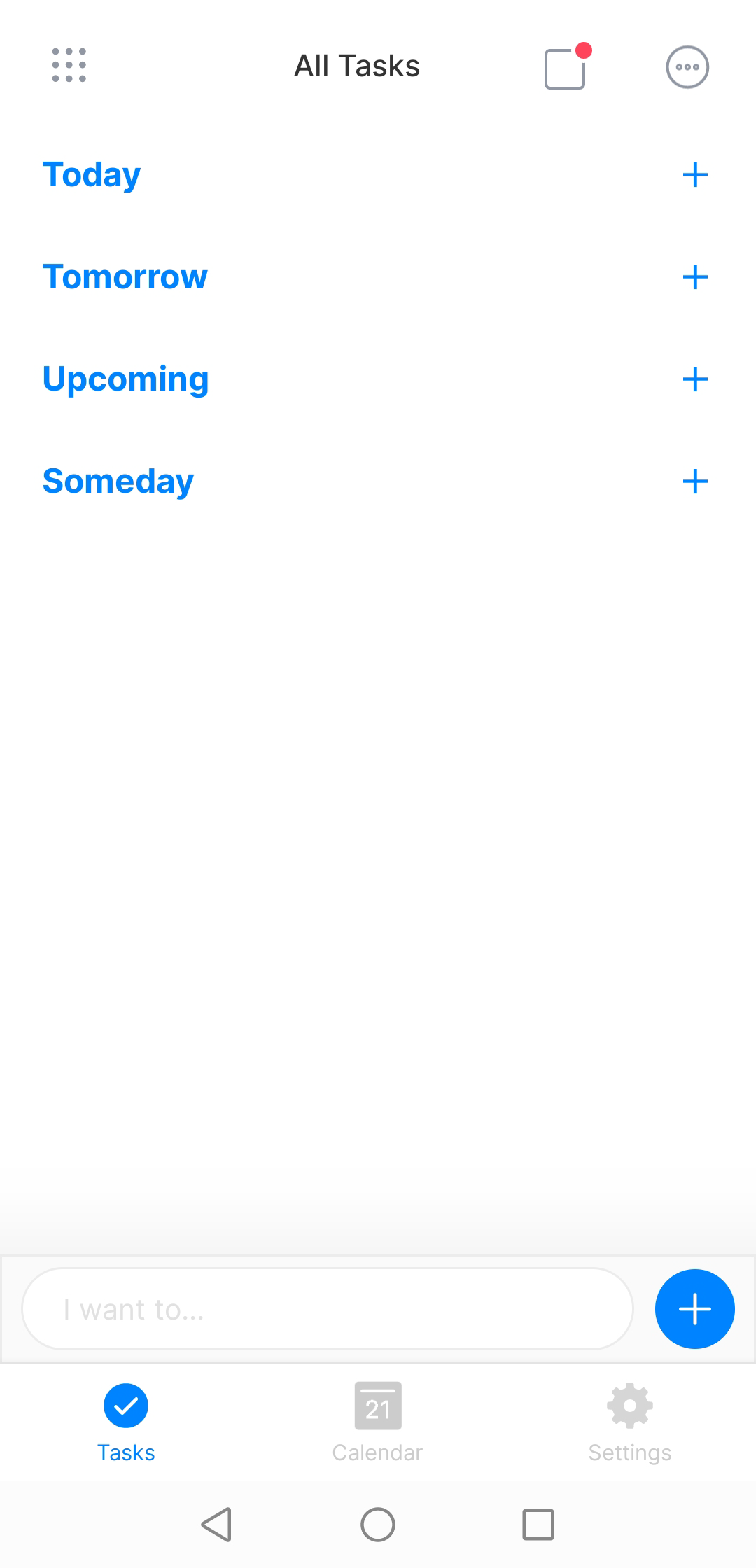The image is a detailed screenshot of a task management application on a smartphone. 

At the top left corner, there's an icon featuring a grid of three rows and three columns of dots. In the center of the top section, the title "All Tasks" is displayed in bold black letters. To the top right, an icon of an empty square with a small red circle positioned at its upper right corner is visible. Adjacent to this, there's a circle with three horizontal dots at its center.

Beneath this header, the options "Today," "Tomorrow," "Upcoming," and "Someday" are listed in blue text, each followed by a plus sign.

At the bottom of the screen, there's a search bar labeled "I want to..." in placeholder text. To the right of the search bar, a notable blue circle with a white plus sign sits, likely functioning as a button to add new tasks.

Further down, the navigation bar contains the following items:
- "Tasks," which is highlighted to indicate it is the currently selected item. It is accompanied by a blue circle containing a white check mark.
- "Calendar," positioned in the middle with a calendar icon above it.
- "Settings," located on the right with a gear icon above it.

Lastly, a set of standard navigation icons is located at the very bottom: a left-pointing arrow, a circle, and a square.

The screenshot is purely interface-focused, with no photographic elements or depictions of people, animals, plants, flowers, trees, or automobiles. The design appears clean and functional, emphasizing task management features.